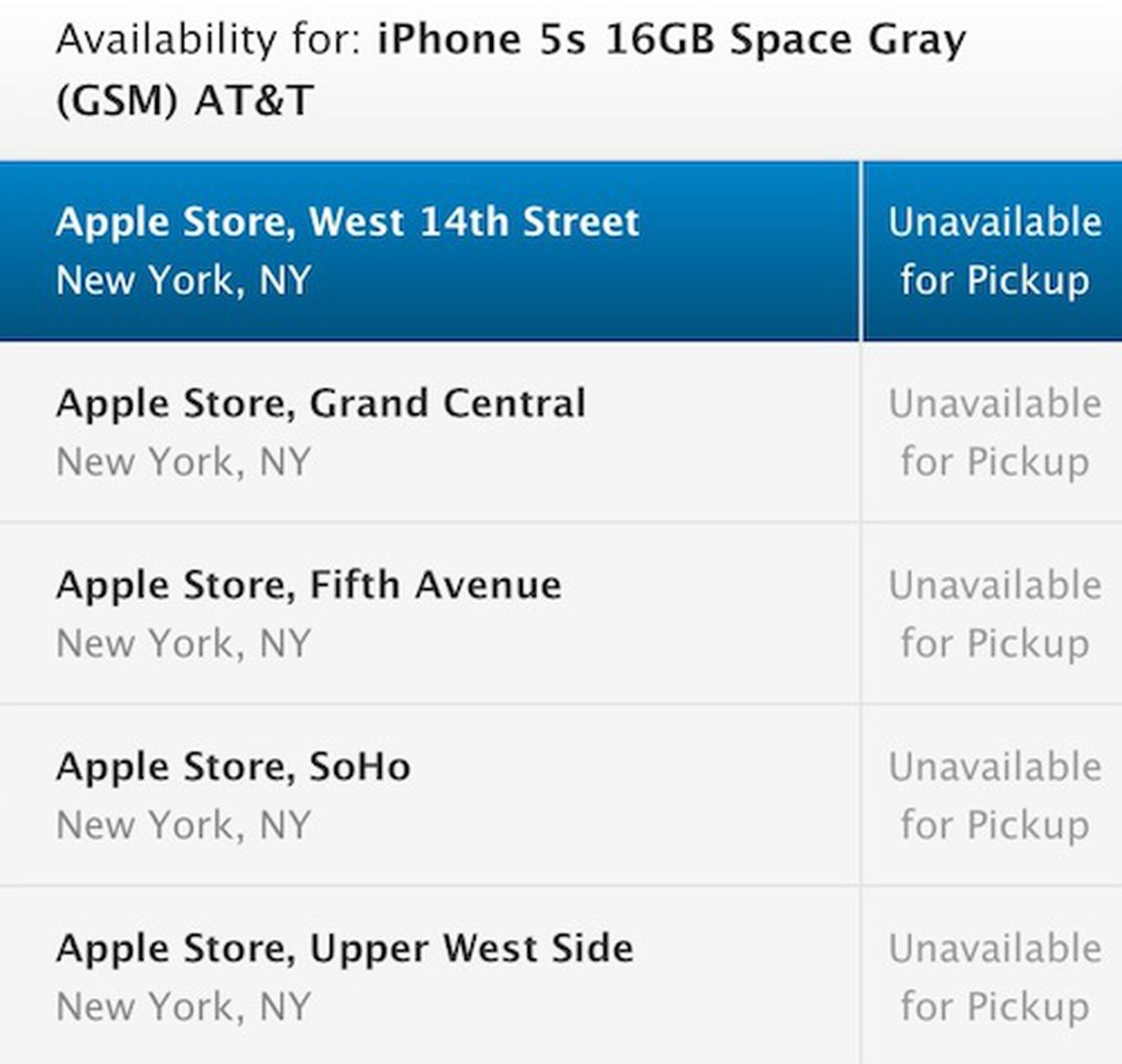A detailed screen capture shows a largely printed website indicating the availability status of an iPhone model. At the top, the website displays "Availability: 4" prominently. Below, in bold black font, it specifies the product: "iPhone 5S, 16 GB, Space Gray," with "GSM AT&T" noted in parentheses. Further down, in blue text, it lists the Apple Store locations in New York along with the product's availability status.

- Apple Store, West 14th Street, New York, NY - A small blue box next to the store name reads "Unavailable for Pickup."
- Apple Store, Grand Central, New York, NY - Marked "Unavailable for Pickup" in gray text.
- Apple Store, Fifth Avenue, New York, NY - Also stated as "Unavailable for Pickup" in gray.
- Apple Store, Soho, New York, NY - Noted as "Unavailable for Pickup" in gray.
- Apple Store, Upper West Side, New York, NY - Similarly marked "Unavailable for Pickup" in gray.

The screen reveals that the user was checking the availability of the iPhone 5S at these specific New York locations and found that it was unavailable for pickup at all of them. The website does not provide options for online orders or a feature to scroll to other stores within New York. The information presented solely lists the out-of-stock status at these specific Apple Stores.